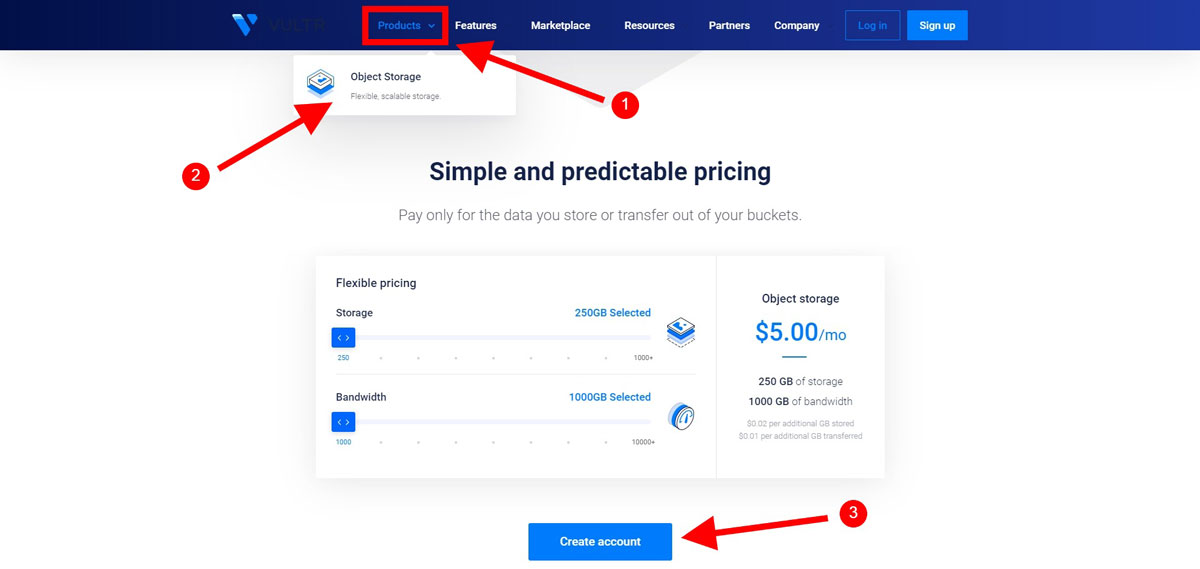Here is a cleaned-up, detailed caption for the image:

"This is an informative webpage designed for purchasing online cloud storage services. At the top, there's a blue navigation bar with a deeper blue tab labeled 'Products,' which is highlighted and bordered in red with the number '1'. Other navigation options in white include 'Features,' 'Marketplace,' 'Resources,' 'Partners,' and 'Company.' There's also a faded dark blue login link and a sign-up button with white text on a bright blue background. 

The central part of the page features details about the 'Object Storage' service, described as 'flexible, scalable storage,' paired with a red arrow marked number '2.' It emphasizes 'Simple and predictable pricing,' where users only pay for the data stored and the bandwidth used. Examples include a storage option for 250 GB at $5 per month and a bandwidth option for 1000 GB.

At the bottom of the page, there is a red arrow labeled '3' pointing towards a 'Create Account' button. The background of the entire page is white, featuring interactive sliders that allow users to adjust their desired storage and bandwidth needs. Overall, the page clearly aims to facilitate the purchasing process for scalable and flexible cloud storage solutions."